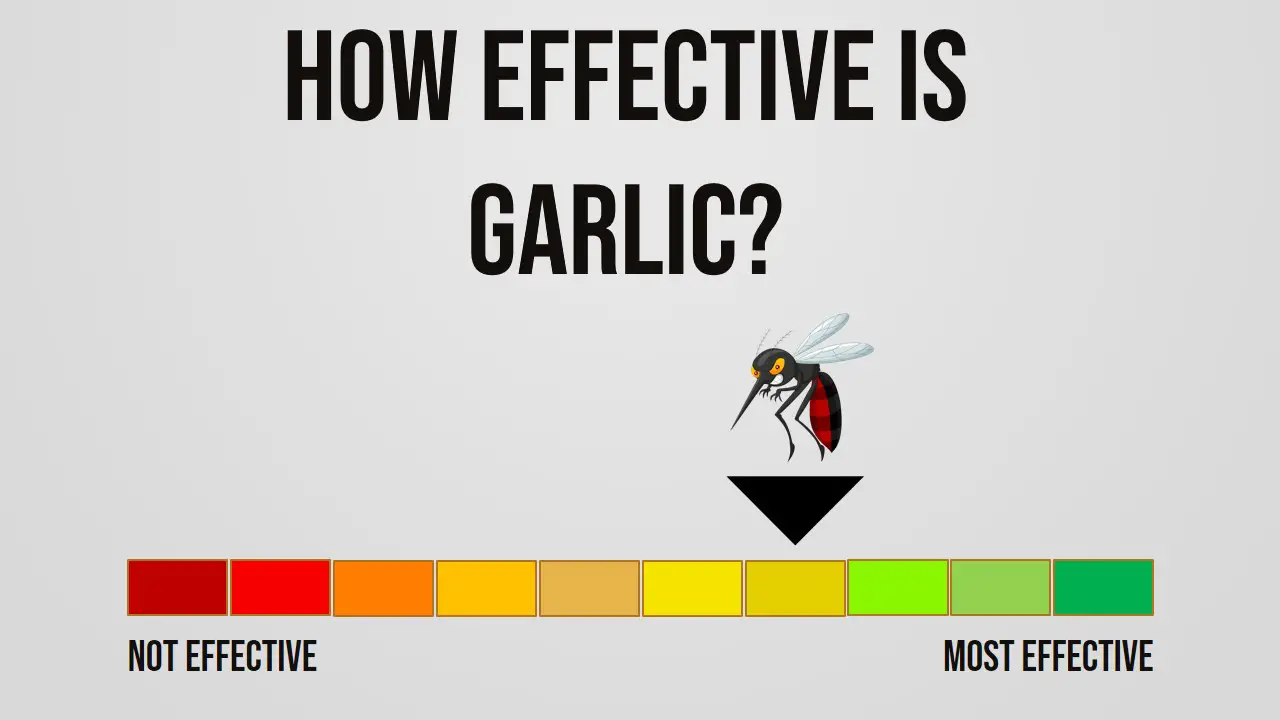The image is an informational graphic with a gray background that asks "How effective is garlic?" in black text. Below the question, there is a horizontally-oriented colored scale, ranging from "Not effective" on the left to "Most effective" on the right. The scale transitions through a spectrum of colors: dark red, deep red, lighter red, orange, orange-yellow, yellow-brown, yellow, yellow-green, green, and two darker shades of green. 

Positioned above the seventh rectangle, which is a yellow color (three from the most effective end), is a black mosquito with clear wings, yellow eyes, red pupils, and a plaid pattern on the underside of its tail. An arrow under the mosquito points to this yellow section on the scale, indicating that garlic is moderately effective. There are no photos in the graphic; everything is illustrated, with clear black text labeling the effectiveness at both ends of the scale.